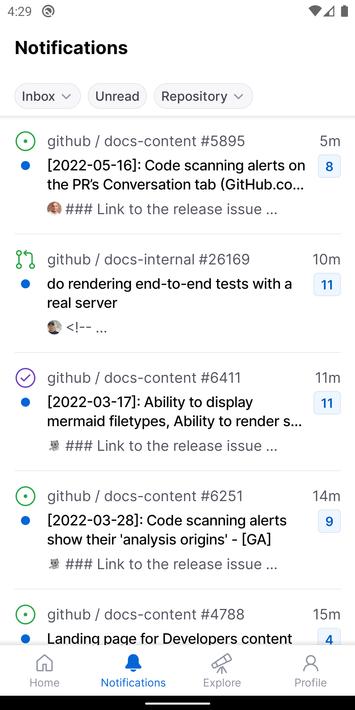The image is a screenshot capturing a notifications page within a mobile app. The context indicates it is from a phone, as evidenced by the time displayed at the top left corner, which reads 4:29, and the battery icon at the top right corner showing a full charge with a completely black battery icon.

Beneath these indicators, the heading "Notifications" is displayed prominently in black text. Directly below this heading are three tabs: "Inbox," "Unread," and "Repository." The "Notifications" tab is currently selected, highlighted in dark blue.

The notifications list below is as follows:

1. **Notification from GitHub**: "Code scanning alerts on the PRs conversation tab" – Received 5 minutes ago.
2. **GitHub Notification**: "Do rendering end-to-end tests with the real server" – Received 10 minutes ago.
3. **GitHub Notification**: "Ability to display mermaid file types and render S... " – Received 11 minutes ago.
4. **GitHub Notification**: "Code scanning alerts show their analysis origins GA" – Received 14 minutes ago.
5. **Partial GitHub Notification**: "Landing page for developers content..." – Received 15 minutes ago.

At the very bottom of the app interface, there is a navigation bar featuring four tabs: "Home," "Notifications" (currently selected), "Explore," and "Profile."